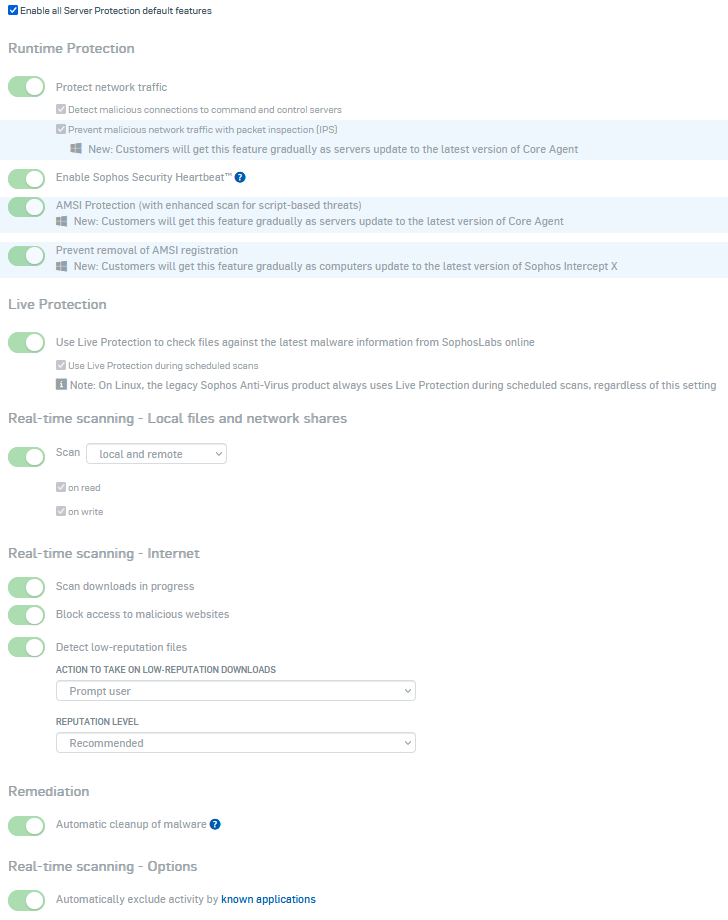In this blurred screenshot set against a white background, various security features and their corresponding toggle buttons are detailed. In the upper left corner, a blue box with a white check mark is visible. To its right, dark gray text reads, "Enable all server protection default features." Beneath this, larger bold light gray text states, "Runtime Protection."

On the left side of the image, a series of toggle buttons are listed vertically. The first toggle, labeled "Protect Network Traffic," is activated and displayed in green. Below it, another toggle is labeled "Enable Sophos Security Heartbeat," accompanied by a small blue circle with a white question mark to its right; this toggle is also turned on. Further down, a toggle for "AMSI Protection" is switched on, followed by "Prevent Removal of AMSI Registration," which is also activated.

The section below is headed "Live Protection," with its toggle turned on. To the right of this toggle, explanatory text states, "Use Live Protection to check files against the latest malware information from Sophos Labs Online."